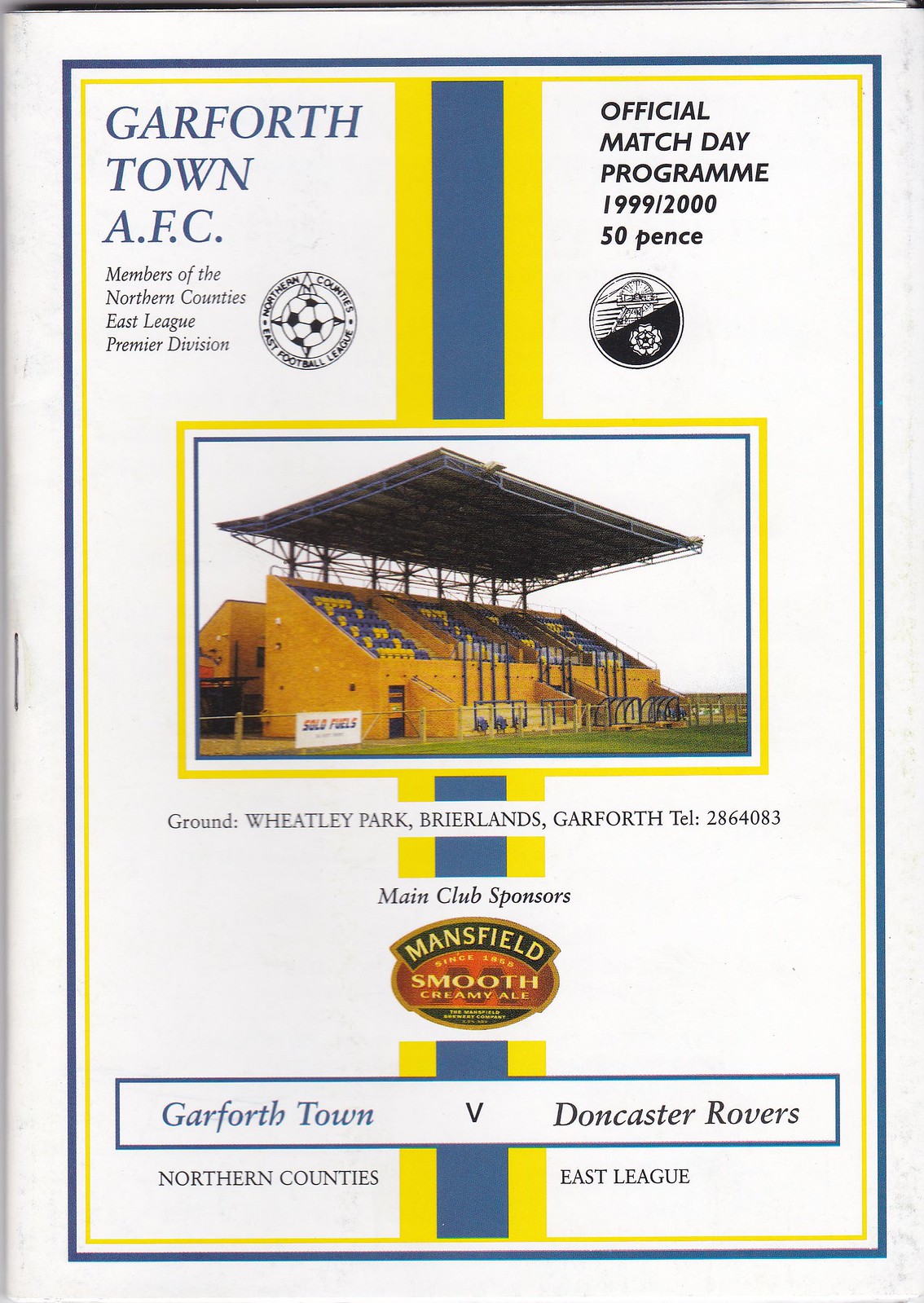This image is of an old soccer program cover from Garforth Town AFC, a member of the Northern Counties East League Premier Division. Dominating the top portion in blue lettering are the words "Garforth Town AFC," followed by the text "Members of the Northern Counties East Premier League Division" in black. To the right, adjacent to a soccer ball insignia, it reads "Official Match Day Program 1999-2000, 50 Pence". Centred in the middle of the program is a photograph showcasing the spectator stand of Wheatley Park, Brearlands, Garforth, where fans sit to watch the games.

The program's background includes a vertical stripe, composed of yellow on the outer edges and dark blue in the centre, running from the top to the bottom of the page. At the bottom, there is a white horizontal strip intersecting the coloured stripe, inscribed with "Garforth Town vs Doncaster Rovers, Northern Counties East League". Below the spectator stand image, it lists "Main Club Sponsor" next to the logo of Mansfield Smooth Creamy Ale, a detail embedded within a brown oval with yellow text. The diverse color palette featuring black, white, blue, yellow, orange, red, and green enhances the vintage aesthetic of the program cover.